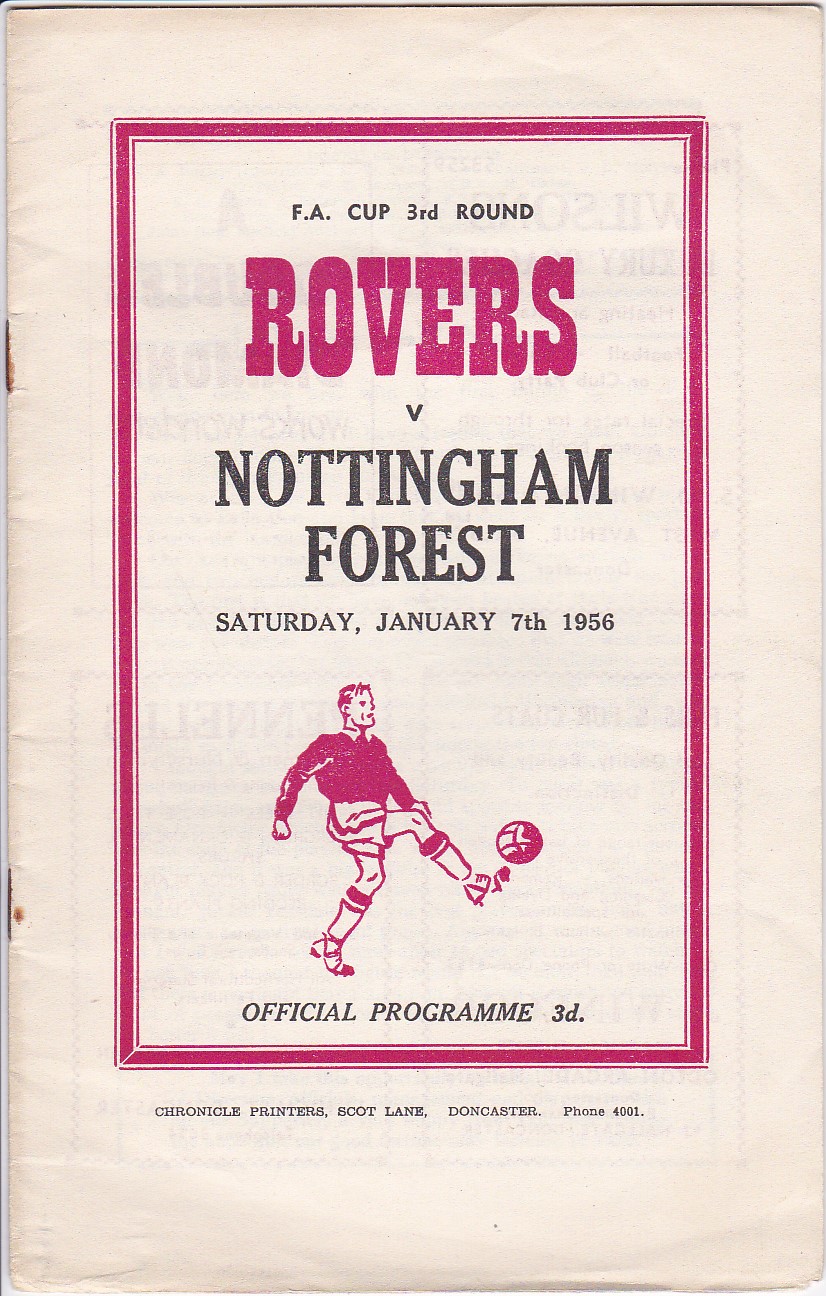The image is a color scan of a vintage football program from Saturday, January 7th, 1956. The front cover, which appears to be made of thin, faded white paper with a pinkish hue and slightly rusted staples on the left edge, prominently features a fuchsia-colored text box. Inside the box, in bold fuchsia font, it reads "FA Cup Third Round: Rovers vs. Nottingham Forest," followed by the date in black font. Below this text, there's an illustration of a soccer player in a fuchsia shirt and white shorts, socks, and shoes, kicking a fuchsia and white soccer ball. The text, also in black, denotes "Official Program 3D" – referring to the pre-decimal British currency price. Outside the text box, along the bottom, it says, "Chronicle Printers, Scott Lane, Doncaster, Phone 4001."